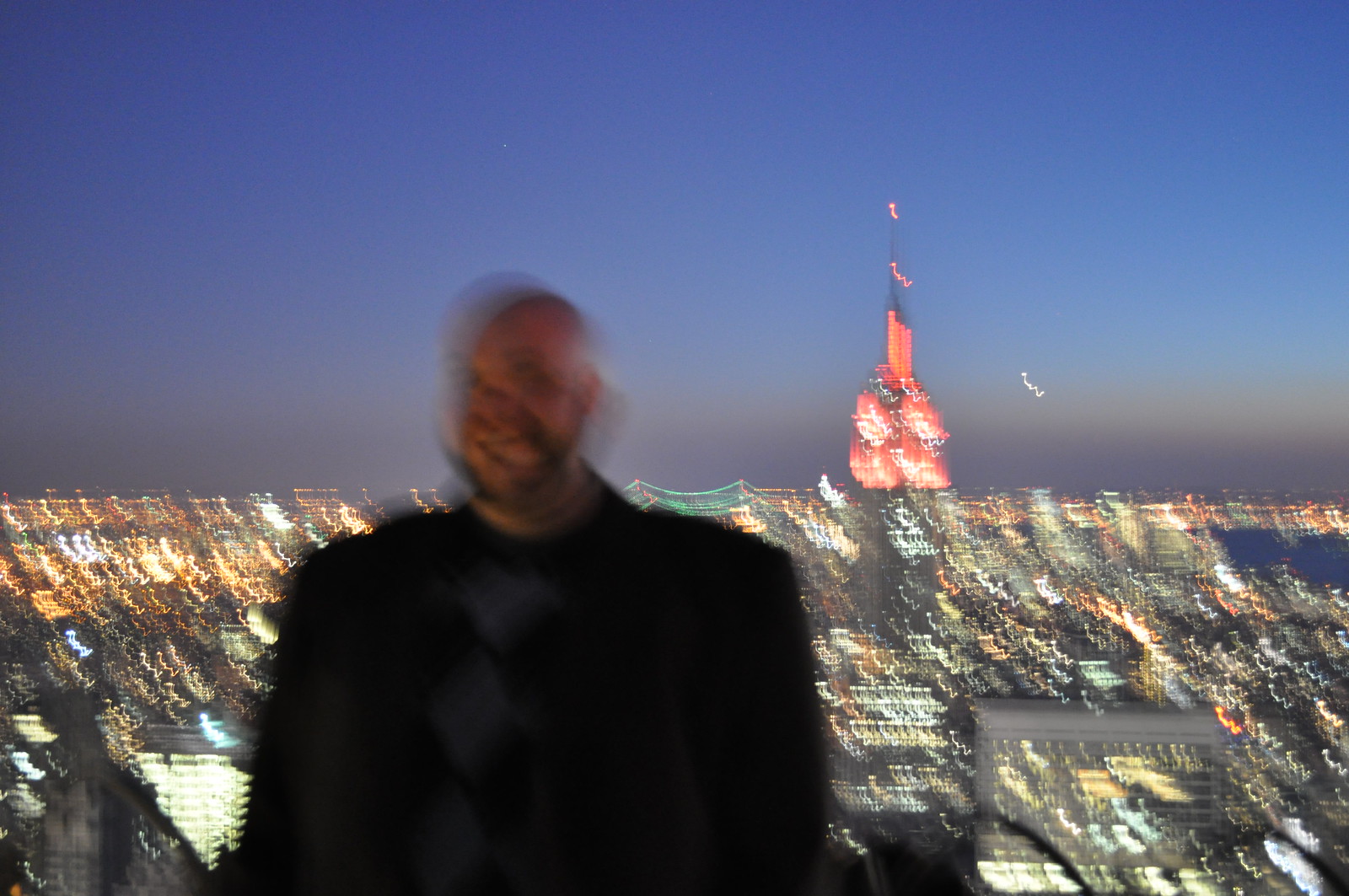The photograph captures a night-time cityscape that is likely New York City, distinguished by the iconic Empire State Building adorned with red lights at its peak. The image is a long-exposure shot, causing every element, including the twinkling lights of buildings and bridges, to appear as streaky, zigzagging lines. The deep navy-blue sky stretches across the top of the image, framing the scene. In the foreground stands a man in a black suit with gray diamond-like patterns on his shirt. His bald head, slight mustache, and short beard are visible despite the overall blurriness. The photograph, taken from a high vantage point, perhaps the top floor of a building, aims to capture him against the backdrop of the illuminated cityscape, possibly as a tourist keepsake. The man's face is extremely blurred, giving the impression of movement during the capture, which adds to the surreal quality of bright, swirling lights in the background. The combination of vibrant city lights and the man's indistinct features create an intriguing and dynamic image.